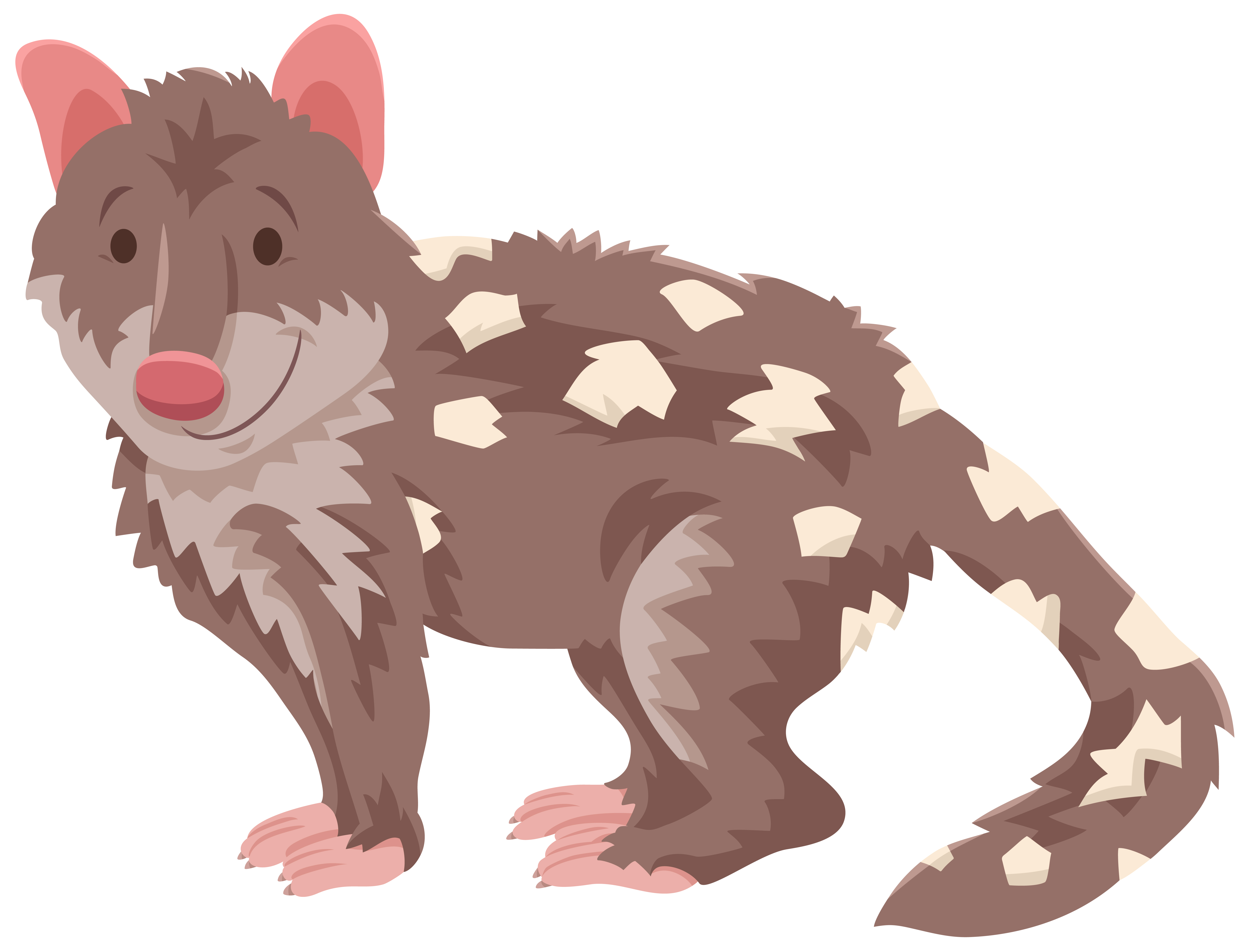This horizontal, cartoon drawing features a unique, cat-like creature that defies typical feline appearances. The animal, mostly adorned in shades of brown and gray, possesses a playful yet curious expression, looking directly at the viewer with its black eyes and smiling with a closed mouth. It has pink, pricked-up ears and a pink nose. The face is predominantly brown, with a lighter area surrounding the mouth. The creature's fur transitions into a lighter brown down the chest and continues with irregular yellow or white splotches along its back and extending to the long tail, which reaches the ground. The tail itself exhibits a mixture of brown, light brown, and darker patches. Adding to its whimsical appearance are its human-like hands and feet, which are also pink with distinct long toes and claws. The creature is depicted on its haunches with both hands and feet touching the ground, suggesting a state of readiness or motion. The image lacks an external border, with a plain white background highlighting the detailed coloration and imaginative design of the creature.